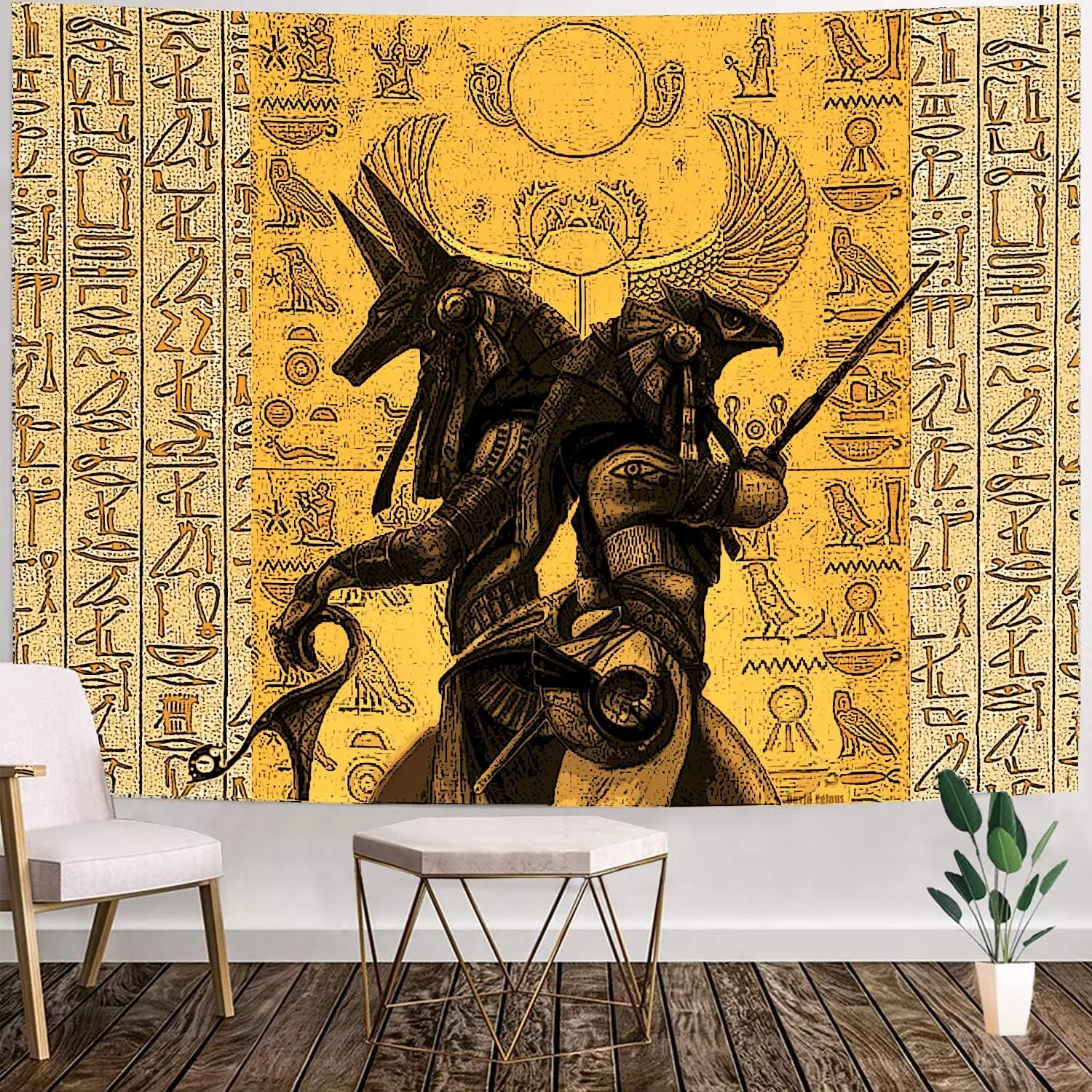This is a high-resolution, professional-quality photograph capturing an elegantly styled room. The room features a pristine white wall adorned with a large, striking golden-yellow image of Egyptian hieroglyphics running vertically across almost the entirety of the wall, except for the bottom one foot. Centered within this backdrop is an even more golden square panel containing additional hieroglyphics and an engraved black eagle. Dominating this central panel are two back-to-back figures dressed in traditional Egyptian attire—one with a wolf mask and an upward-pointed sword, and the other with an eagle mask holding what appears to be a staff with a swirling, almost closed circle handle. 

In the foreground, the room boasts a dark wooden plank floor. Positioned to the left is a light wood and light beige cloth armchair, paired with a stylish matching table that features a light gold metal wire support frame and a possibly marble white top. On the right side of the room stands a white pot holding a green plant, contributing a touch of life to the sophisticated setting. This detailed photograph skillfully blends ancient Egyptian art with modern interior design elements, creating a visually engaging and culturally rich scene.